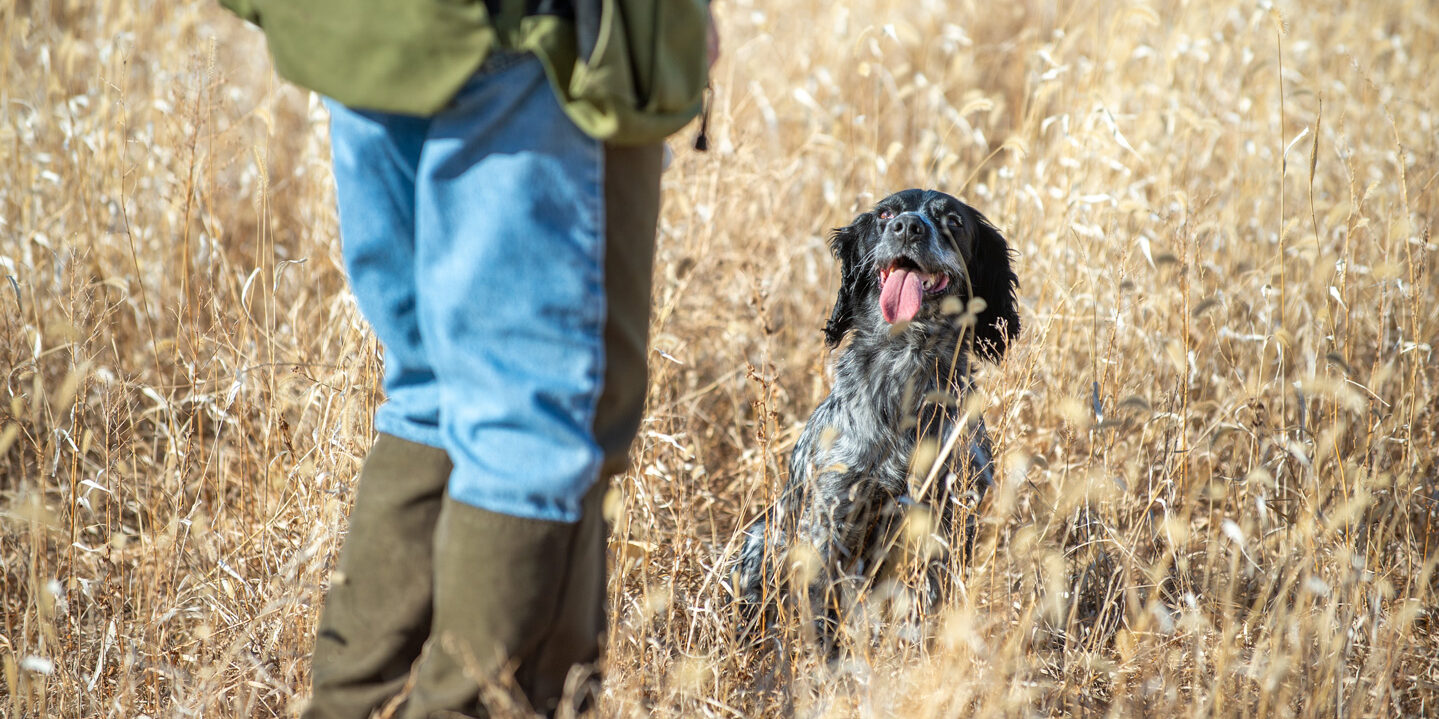The image captures a scene in a sunlit field of tall, dry, light brown crops, possibly wheat, with a person and a dog. The person, whose upper body is mostly out of view, is wearing blue jeans, olive green boots, and the bottom of a green jacket is visible. They appear to have their hands in their pockets. The field seems expansive and lifeless, with tan, high grasses that could suggest an agricultural landscape. In front of the person sits a dog with a mostly black face and a mixed black and white coat. The dog, which appears to be a medium-sized hunting breed, is gazing up at its owner with its tongue hanging out and ears back, exuding a cheerful demeanor. The scene suggests a moment of companionship in a quiet, rural setting, possibly part of a hunting excursion or a countryside walk.